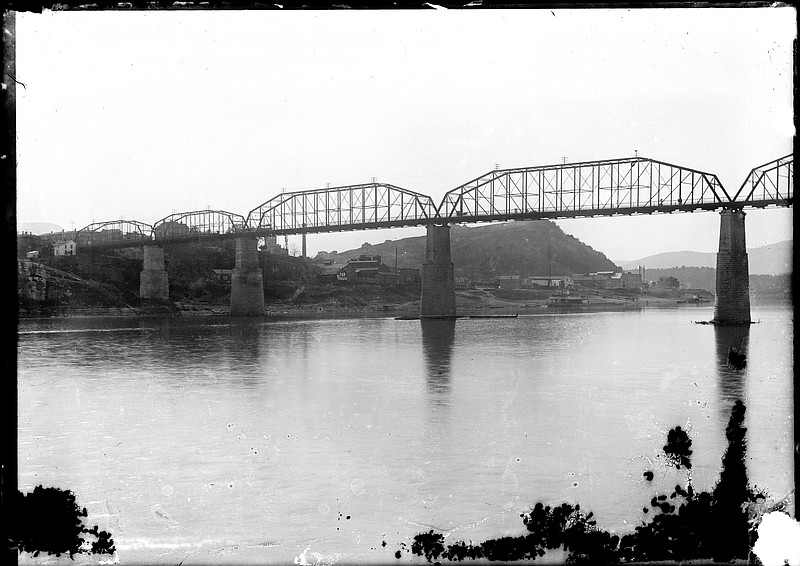This is a black and white photograph with a worn, black-colored border and some damage in the form of black spots near the bottom corners. The image captures an outdoor setting featuring a large river, calm and expansive, with an industrial-style metallic bridge spanning over it. The bridge is distinctive, supported by tall, tapered concrete pillars, with steel girders forming elongated arches and a guardrail along its sides. Below the bridge, the river flows serenely, lined with several low industrial buildings on the near shore. These buildings, adorned with steam pipes, present a rugged, utilitarian ambiance. The land appears uneven and rises into steep hills or slag heaps in the background, possibly indicative of a mining or quarrying operation. The sky above is a light, featureless white, enhancing the stark contrast of the black and white palette.